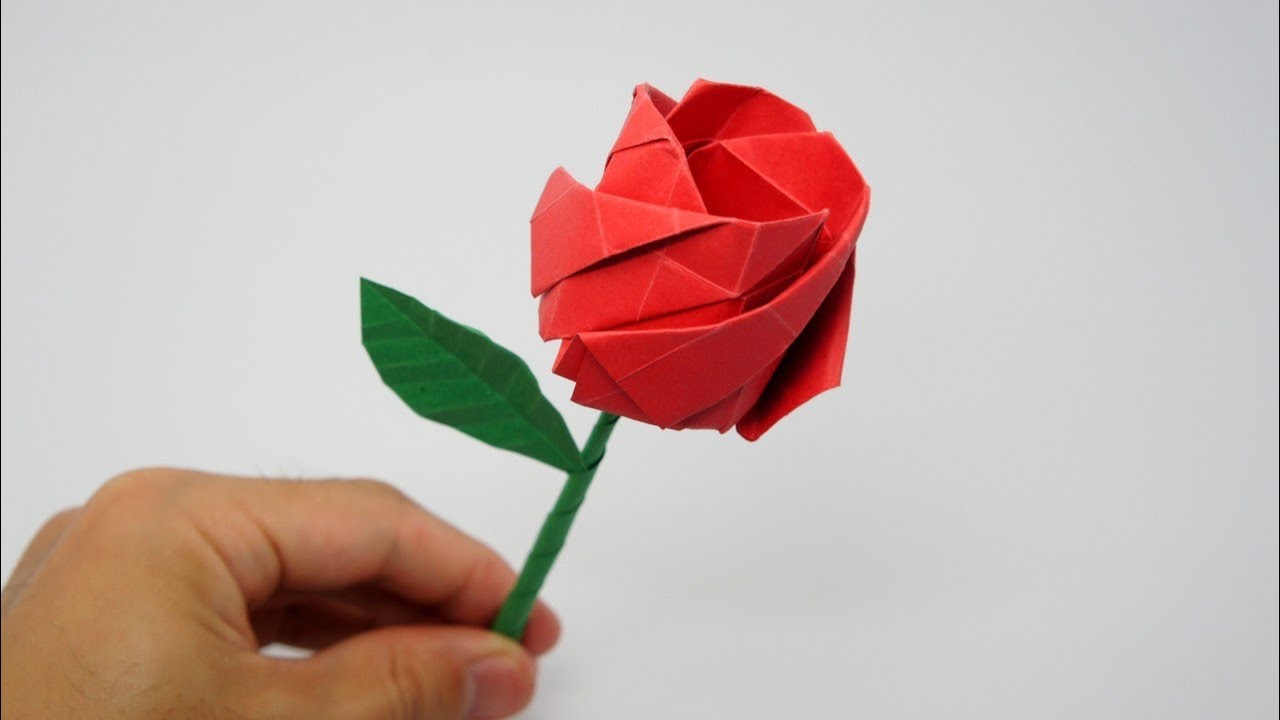This image showcases an intricate origami rose crafted from red paper, held delicately by a light-skinned left hand. The detailed creases and numerous folds, both rectangular and triangular, captivate attention, revealing the meticulous effort taken to shape the rose. The green paper stem, spiraled and robust, supports the vibrant bloom, complete with a single green leaf extending from the left side. The background is a light gray, providing a subtle contrast that highlights the artistry of the paper flower. The hand, lightly haired and mostly visible in the lower left corner, adds a personal touch to the image, emphasizing the delicate human interaction with the crafted rose.